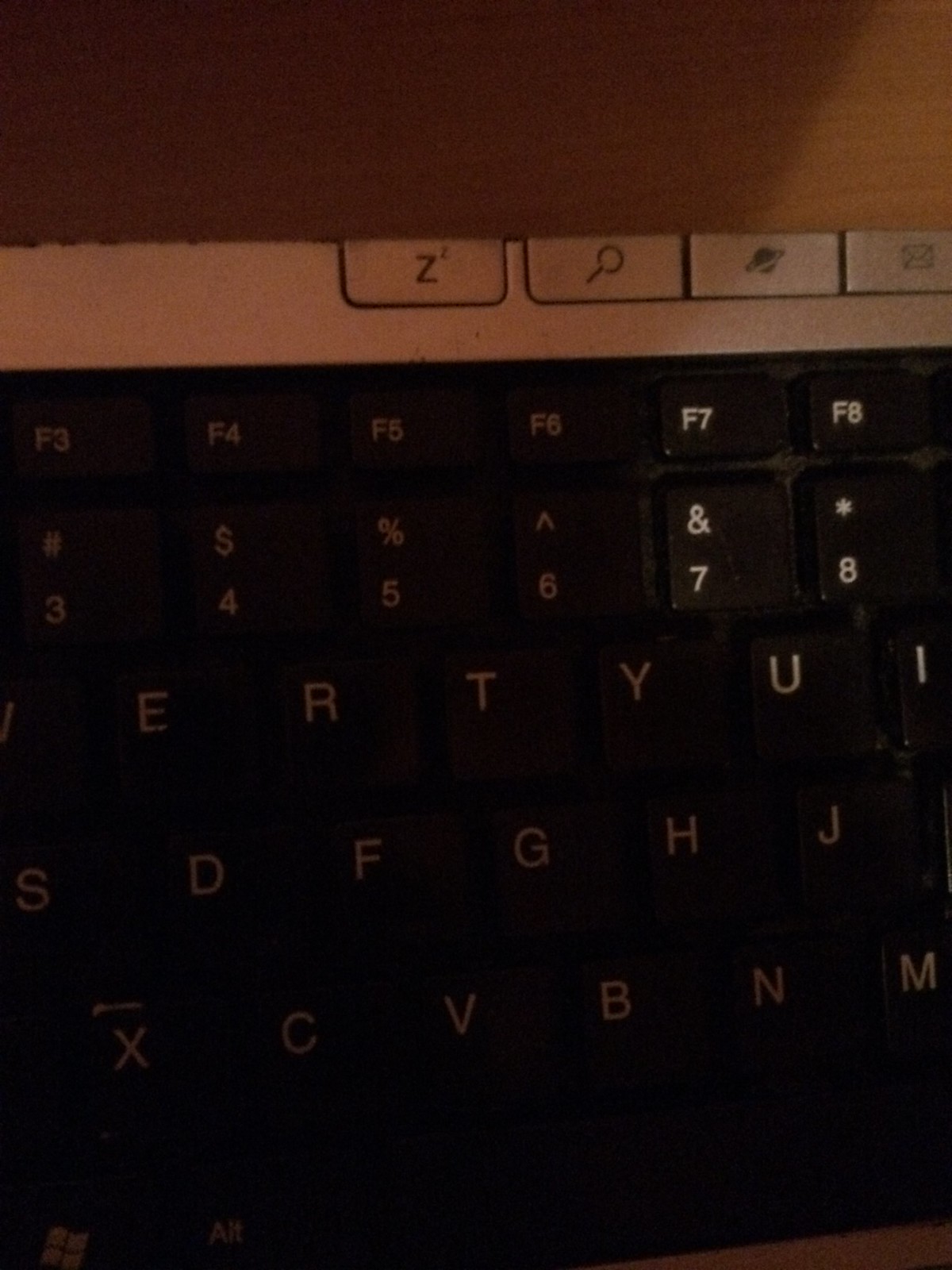This photograph captures a dimly lit, close-up view of a keyboard, likely from a laptop or possibly a tablet, taken in a low-light indoor setting. The focus is on the upper section of the keyboard, prominently featuring the F7 and F8 function keys, along with the number keys 7 and 8, bearing the symbols & and * respectively. The clearly lit letter keys U and I stand out amidst the shadows engulfing the other keys. 

A silver metallic band spans the very top of the keyboard, housing an array of four distinct buttons adorned with pictograms: a "Z" with a superscript "1," a magnifying glass, a planet, and an envelope icon. These buttons provide additional functionalities. Below the silver band lies a row of function keys extending from F3 to F8. The visible portion of the keyboard continues to show letter keys ranging sequentially from S to J, and further down from X to M, and E to I. 

Just beneath the keyboard, a sliver of brown wooden desktop is noticeable, suggesting the keyboard rests on a desk. The overall design hints at an older model keyboard with black keys and white lettering, bringing a nostalgic feel to this dimly captured scene.